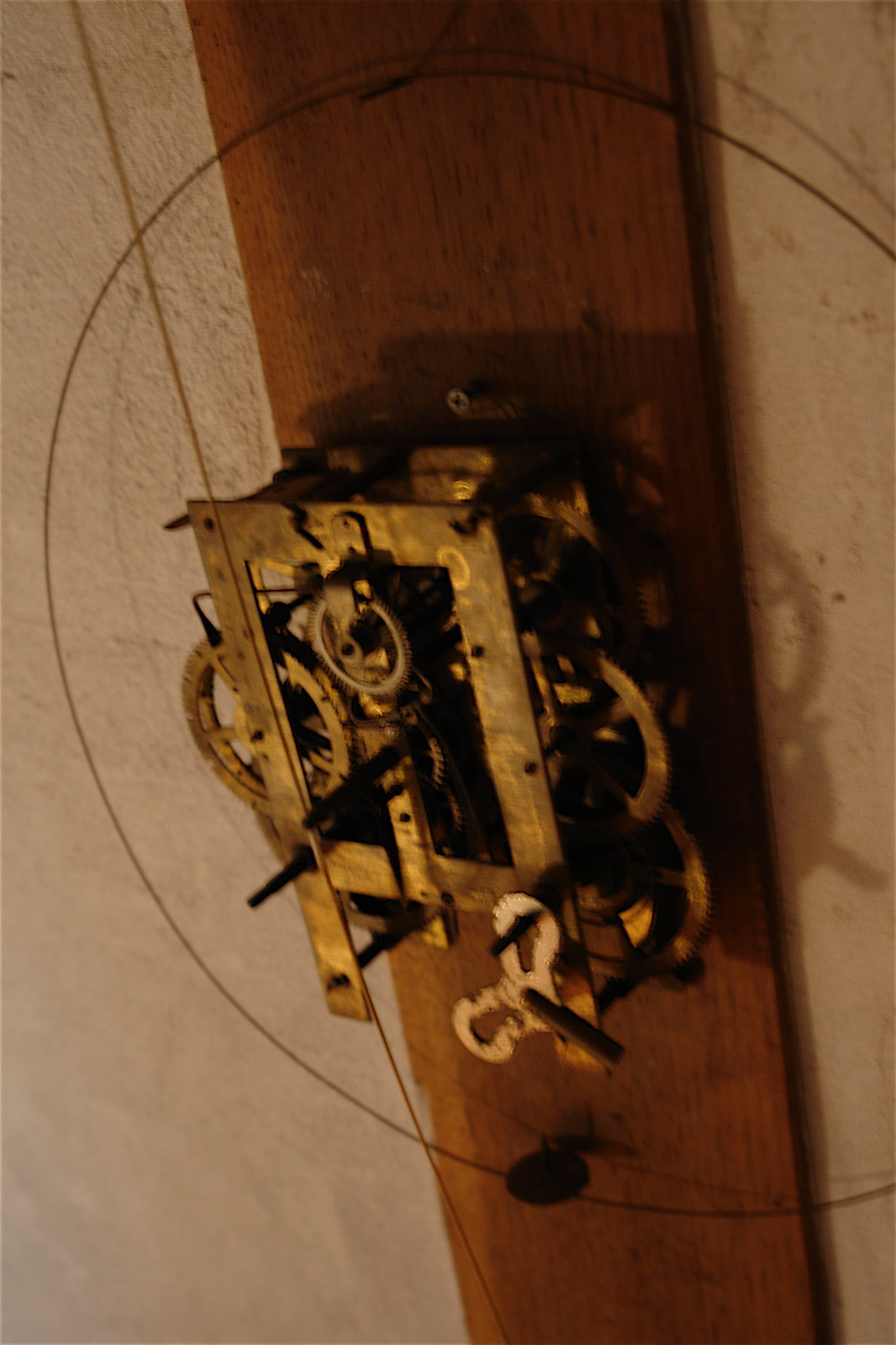A vertical, possibly pine, one-by-six piece of wood is mounted against a brown background. Affixed to the wood is a detailed, brass clock mechanism, prominently featuring a winding key hanging from it. The intricate inner workings, comprising numerous interlocking gears housed within a rectangular brass frame, are visible. The mechanism is topped with a large, clear circular piece, presumably glass, which occupies most of the vertical space but is truncated on the right side, suggesting it might be a clock without its traditional face.